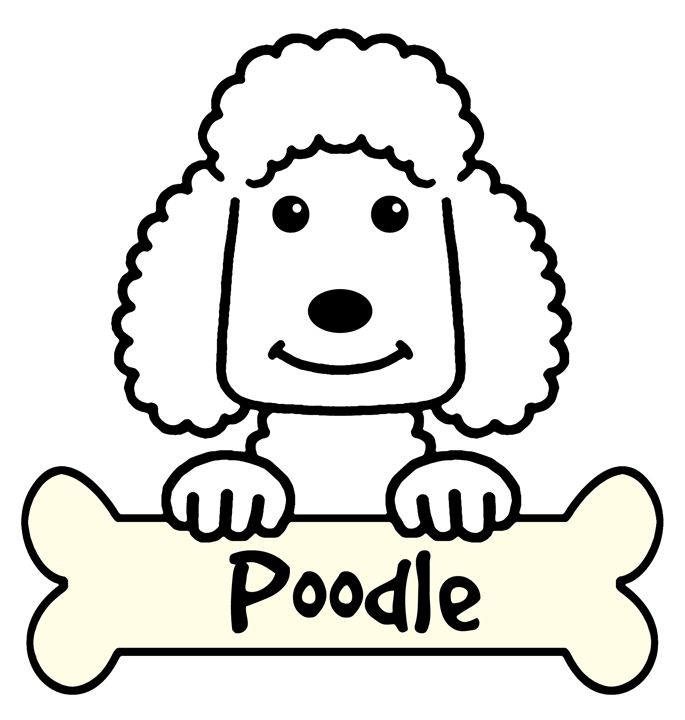This is a detailed cartoon illustration of a happy poodle, depicted in black and white. The smiling poodle, with a prominent button nose and round eyes featuring small white highlights, is facing forward and has its curly top hair clearly visible. The poodle’s front paws rest on a large, off-white or cream-colored bone occupying the bottom third of the image. This bone has the word “poodle” written on it in black. The rest of the dog's body is obscured by the bone, showcasing only its head, neck, and paws. The drawing is outlined in black and has no background, implying a transparent setting. This simple, yet charming, sketch could easily serve as clip art or in an advertisement due to its clean lines and straightforward design.